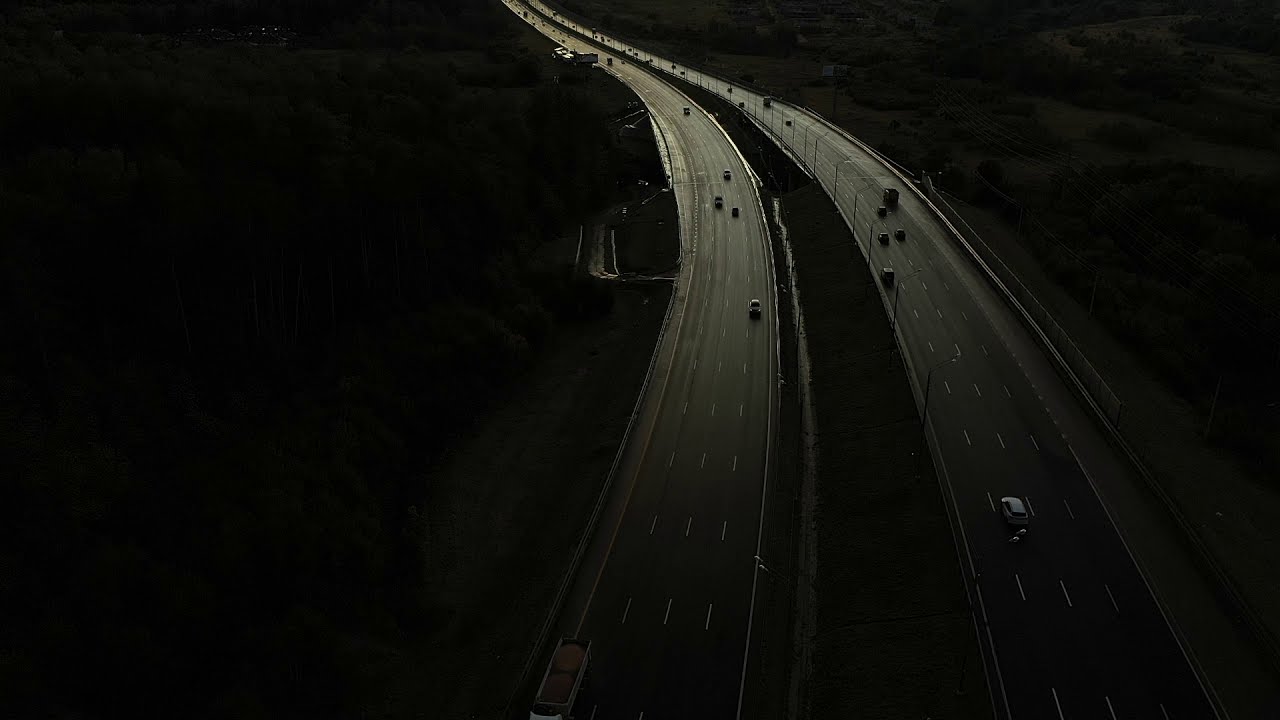This color photograph captures two parallel highway overpasses taken during a time with minimal natural light, possibly near sunset or sunrise. These overpasses, each consisting of four lanes divided by dotted white lines, begin at the lower right of the image and curve gently to the left, ascending a slope as they progress. The road on the right is filled with vehicles moving away from the viewer, including a prominent small white vehicle, whereas the road on the left has traffic coming towards the viewer with a noticeable truck that has two red circles in its bed. The highways are flanked by tall fences in the center and shorter ones on the far right. While the overall scene is shrouded in darkness, the ambient light, likely artificial, faintly illuminates parts of the roads. The surrounding landscape includes an empty area and possible vegetation or trees. There's also a side road or maintenance track briefly running off and rejoining the left highway. The darkness envelops most of the image, rendering the detailed landscape indistinct but hinting at the presence of hills or buildings.